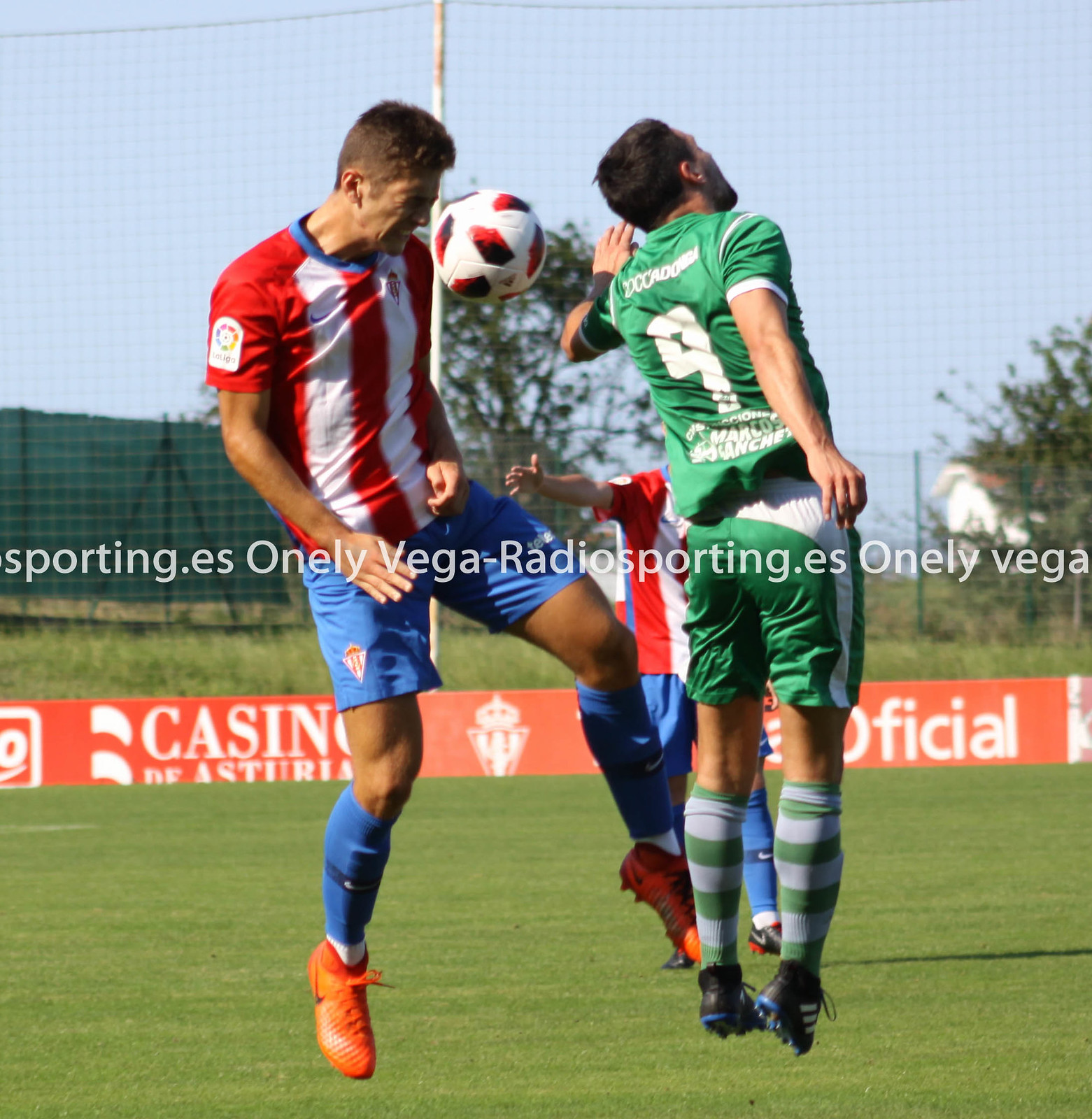This action-packed daytime photograph captures a thrilling moment in a football match. Against a backdrop of a clear blue sky and the sun shining down, three players are the focus on a neatly cut grassy field bordered by banners advertising brands like Casino and Asturias, along with official logos. In the foreground, two players from opposing teams leap into the air, competing to head a soccer ball. On the left, a player in a red and white vertically-striped jersey, blue shorts, and matching blue socks, sporting orange cleats, is caught mid-air with his head tilted forward, seemingly about to hit the ball with his forehead. His short brown hair and intense grimace are clearly visible. To his right, a player in a green kit with the number nine on his back, complemented by green shorts, green and gray horizontally-striped socks, and black cleats, is also airborne. His back is towards us, his left arm bent at the elbow and raised slightly, and his right arm trailing behind. His head, covered in dark hair, is slightly tilted back. Between them, further in the background, another player wearing the red and white jersey, blue shorts, and black cleats is seen extending his right arm, but his details are largely obscured. The field is surrounded by green fences and trees, and in the center of the image, text reads "VegaRadioSporting.es" repeatedly. The soccer ball, white with dark blue and red markings, hovers inches from the head of the red-and-white jersey player.